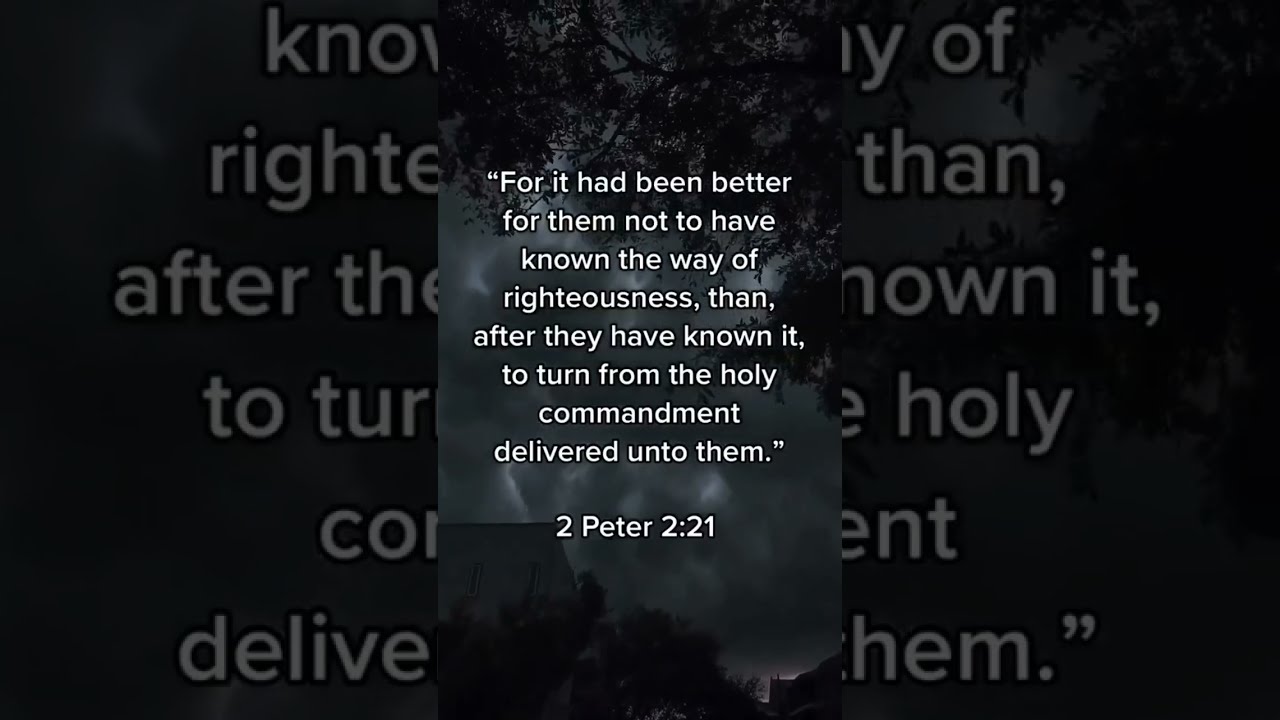The digital image has a dark, black-dominated background that resembles a night sky filled with dark, shadowy clouds. Silhouetted tree branches with foliage stretch across the scene, creating a somber, mysterious atmosphere. In the vertical center of the image, framed like a phone screen, is a white text quote from the Bible, specifically 2 Peter 2:21, which reads: "For it had been better for them not to have known the way of righteousness, than after they have known it, to turn from the holy commandment delivered unto them." The quote is prominently featured against the dark background, evoking a reflective or solemn mood, and in the lower left corner, the faint outline of a rooftop's shingles subtly appears, adding a grounded element to the otherwise ethereal setting.